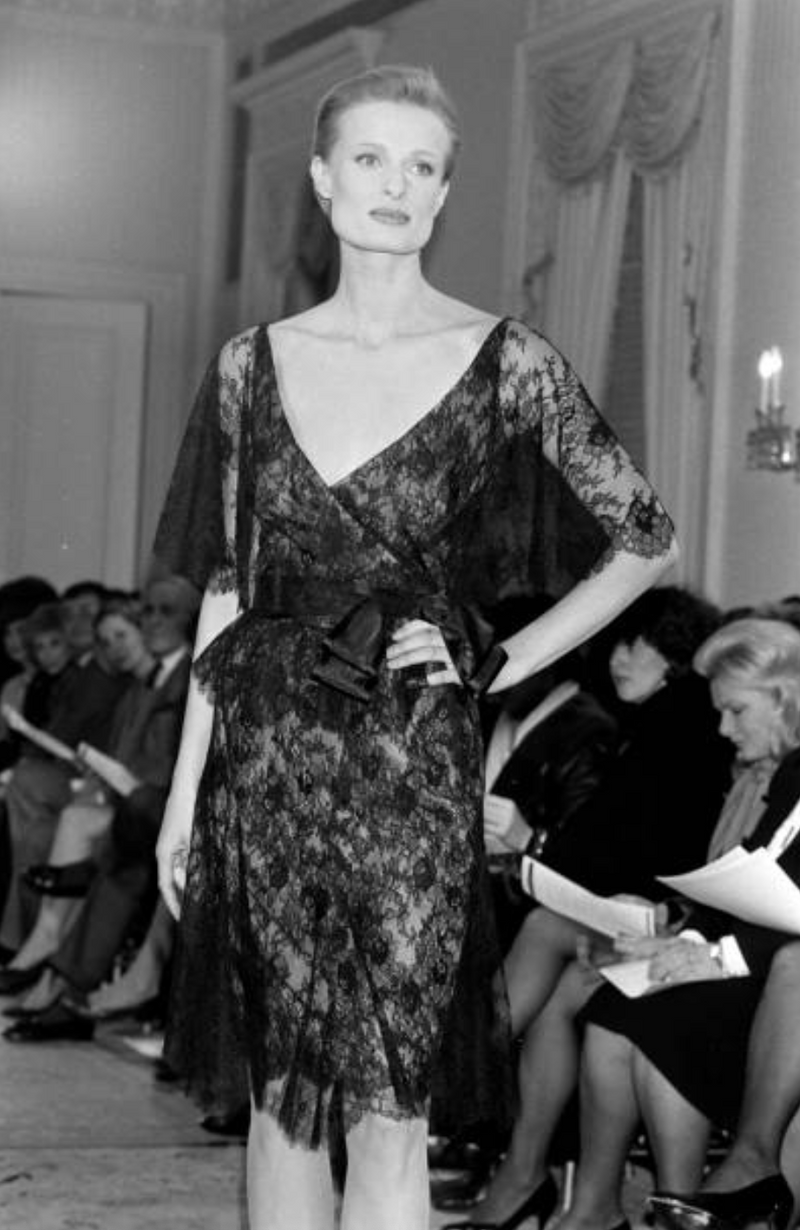This black and white photograph captures a white woman in her late 30s, posing with a model-like confidence. Her short haircut, resembling a men's cut, frames her face as she stands with her left hand on her hip. She dons a dark, almost translucent black lacy dress with a ribbon accentuating her waist. Her stance is firm yet graceful, facing forward with her head slightly tilted to the right, gazing off in the same direction.

Behind her, a group of well-dressed individuals, including both men and women, sit attentively with pamphlets or programs in their hands, suggesting a formal event, possibly a fashion show. The setting is an elegant interior with tall windows adorned with ornate curtains, giving the scene a sophisticated ambiance. The focus remains on the poised woman in the foreground, embodying the essence of classic fashion.